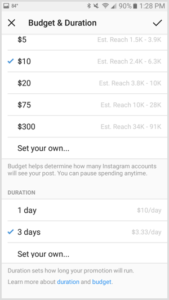This screenshot captures a section of a mobile application's settings interface, set against a grayish-white background. 

At the top left, there are several notification symbols, including an image icon and a temperature reading of 54 degrees. Alongside these are indicators for Bluetooth connectivity, muted volume, Wi-Fi connection, a strong cellular signal, and a battery level at 90%. The time displayed is 1:28 p.m.

Below this bar, on the left, there is an "X" icon next to the labels "Budget" and "Duration," with a checkmark located on the right side. 

The section titled "Budget" presents preset monetary increments: $5, $10 (highlighted with a blue checkmark), $20, $75, and $300. There is also an option labeled "Set Your Own," allowing users to manually input a specific amount.

Below the budget options, under "Duration," users can choose from preset time periods: 1 day, 3 days, or use the "Set Your Own" feature to customize the duration according to their preference.